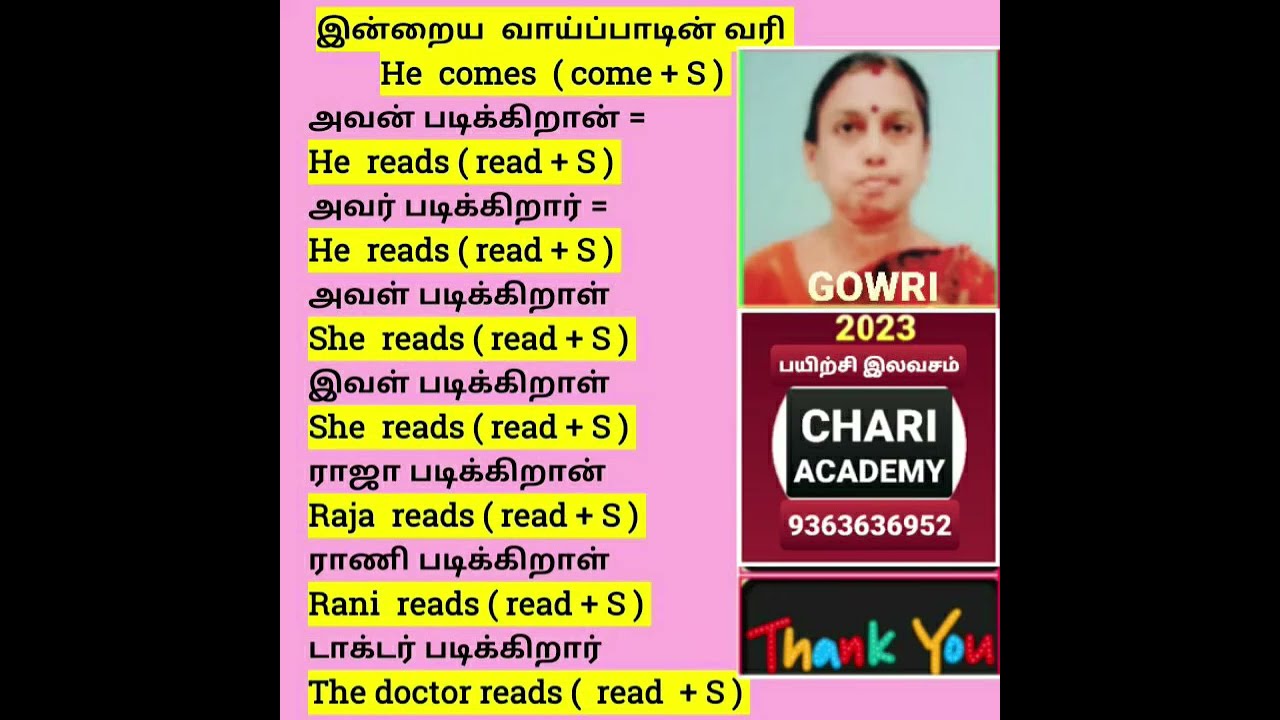The image depicts an Indian woman with dark hair, a bindi on her forehead, and dressed in a red top, centered between two vertical black borders. The picture resembles a mug shot or driver's license photograph. Underneath her image, the name "G-O-W-R-I" and the year "2023" are displayed, followed by unreadable text in a foreign script. Further down, in white capital letters on a black background, it says "C-H-A-R-I-ACADEMY," and below that, on a red background with white text, is a phone number "9-3-6-3-6-3-6-9-5-2" and the words "Thank you" in multicolored fonts. 

To the left of the woman's portrait, the image features extensive text in both a foreign language and English. The text, highlighted in yellow boxes, translates to phrases like "he comes," "he reads," "she reads," "Raja reads," "Rani reads," and "the doctor reads," each followed by “read + capital S” in parentheses. The background of the text area is predominantly pink. This portion of the image appears to be educational, possibly from an online language learning class, with colorful elements including pink, yellow, black, and other hues.